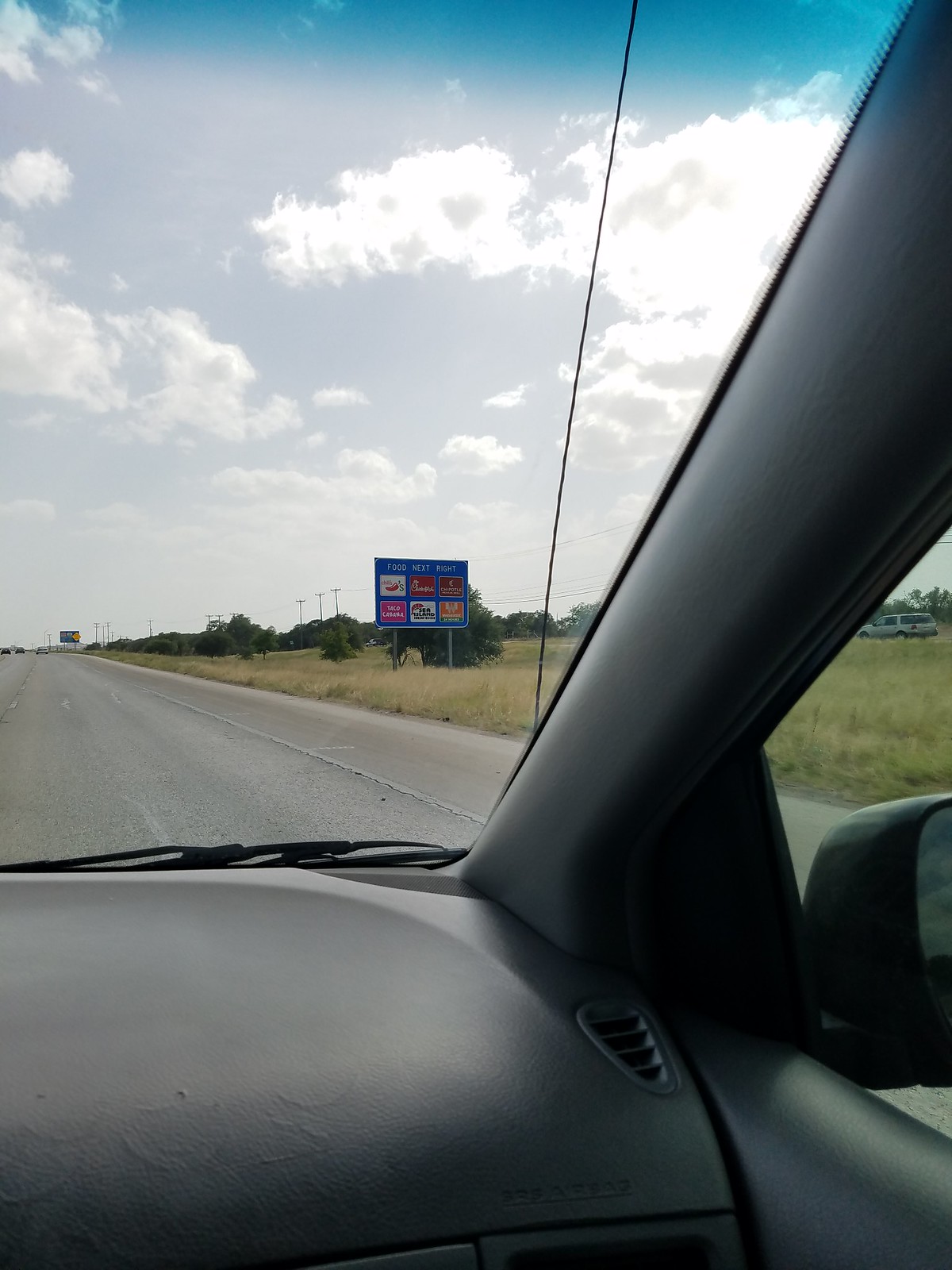The image was captured from the passenger seat of a car traveling in the left lane on a highway. Visible from inside the car are the right side of the windshield, the side mirror, the air vent, and a portion of the windshield wiper antenna. Outside the car, there is an expansive green landscape. A large blue sign on the roadside, although unreadable in detail, displays recognizable logos for Pilot gas station, Chick-fil-A, and possibly Red Roof Inn, indicating nearby amenities at the upcoming exit. The road ahead appears empty, with no other vehicles in sight, adding to the serene atmosphere of the drive.